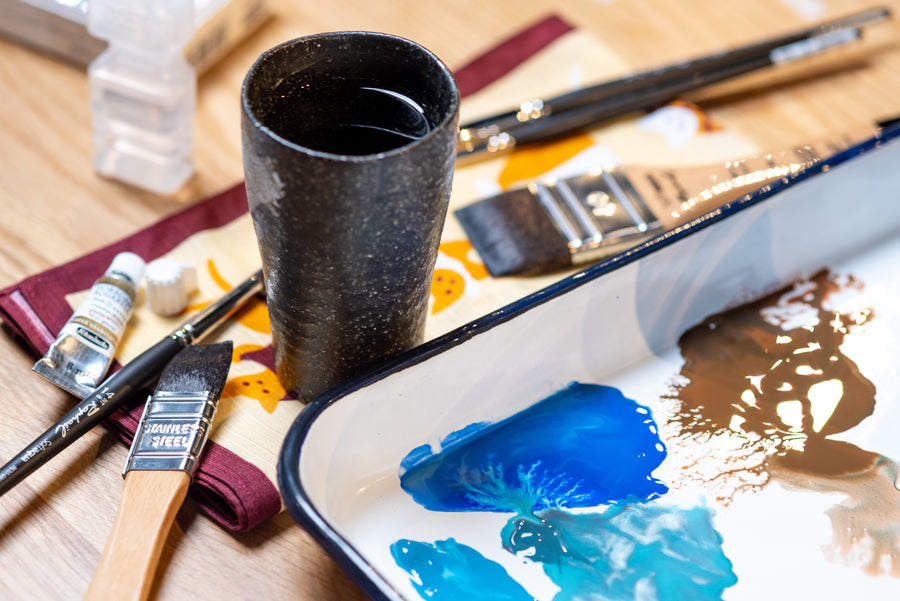This close-up photograph captures a detailed artist's painting setup on a wooden desk. Central to the composition is a sparkly black ceramic cup filled with water, surrounded by various wet paintbrushes of differing thicknesses and lengths. These brushes are resting on a folded cloth napkin with a red border and a patterned design featuring cartoon cats in yellow and gold hues. In the bottom right corner of the image, there's the edge of a white ceramic tray used for mixing paints, displaying smudges of royal blue, light blue, turquoise, brown, green, and pink. A silver tube with a white label and cap is also visible among the painting supplies. The scene is meticulously arranged with the necessary tools for painting, highlighting the organized yet creative nature of the workspace.